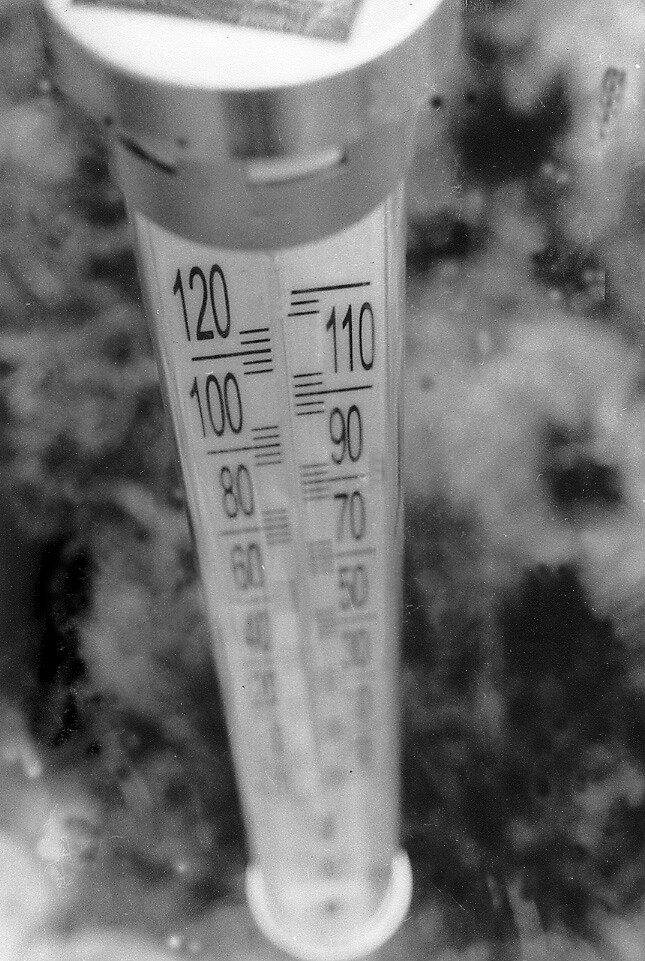The black and white photograph is very blurry and out of focus, making it difficult to discern the background, which appears to be a fabric with an indeterminate design. The image features a variety of shades ranging from white to gray to black, arranged without any specific pattern. Central to the photograph is a cylindrical thermometer, which is encased in glass. At the top of the thermometer, there is a round metal piece with a few holes and grooves. The thermometer has a white background, with legible numbers ranging from 120 down to 30, although the finer details and additional numbers are obscured by the blur. Each main number is separated by five smaller lines, indicating precise temperature measurements. The bottom part of the thermometer is smoothly rounded.